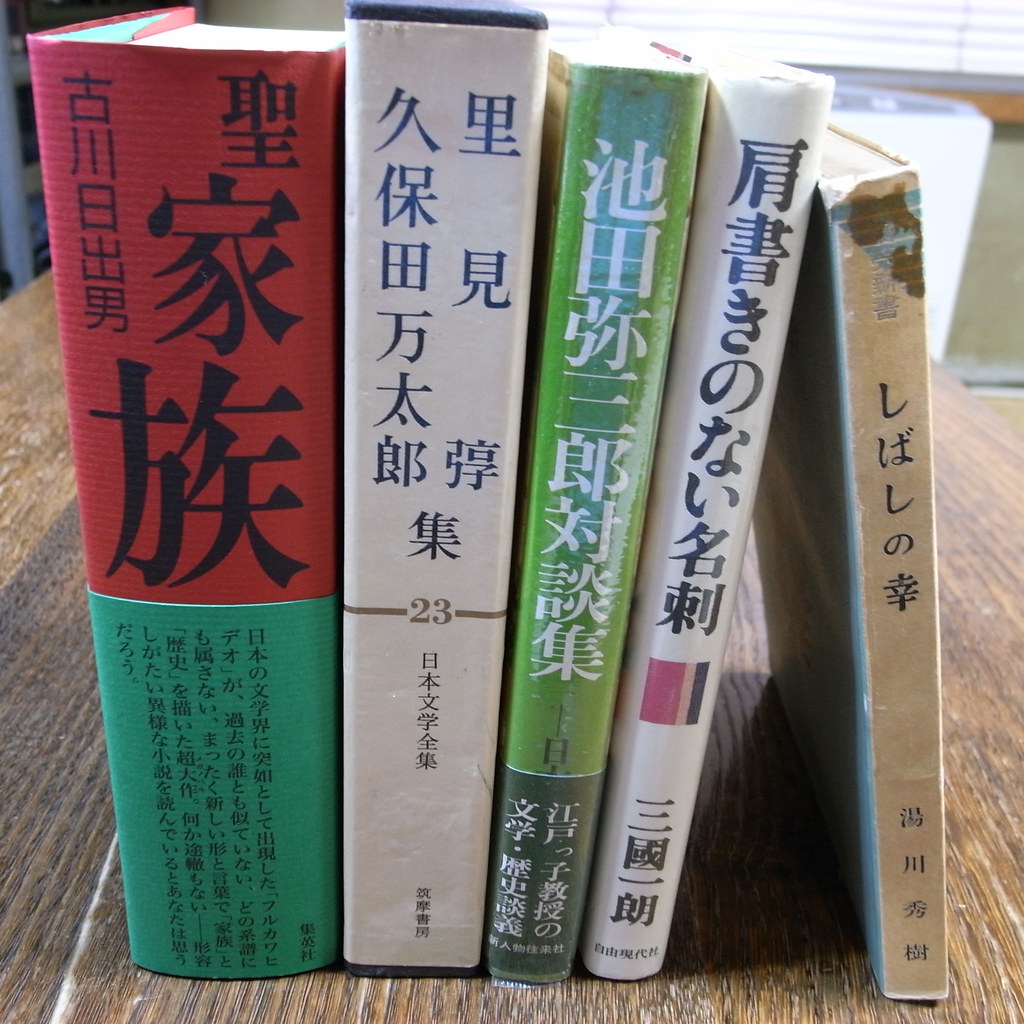In this detailed photograph, five books with spines facing the camera are standing upright on a slightly worn, brown, wood-grained table. From left to right, the first book features a red upper half and a teal lower half with Chinese characters. Next to it, a white book displays blue and black Chinese writing, including a prominent gold stripe labeled with the number '23.' The third book’s spine is divided, with the upper portion in light green and the lower part in dark green, both sections displaying Chinese script. The fourth book in the row has an entirely white spine adorned with a small, colorful emblem a third of the way up, featuring red, light brown, and dark brown sections along with additional Chinese characters. Lastly, the fifth book, slightly inclining towards the adjacent books for support, has a dingy brown spine marked by a stain at the top and six central Chinese characters. The scene is set against a backdrop where a window with brown trim and open blinds is visible in the distance, along with a small glimpse of a gray wall beneath it.